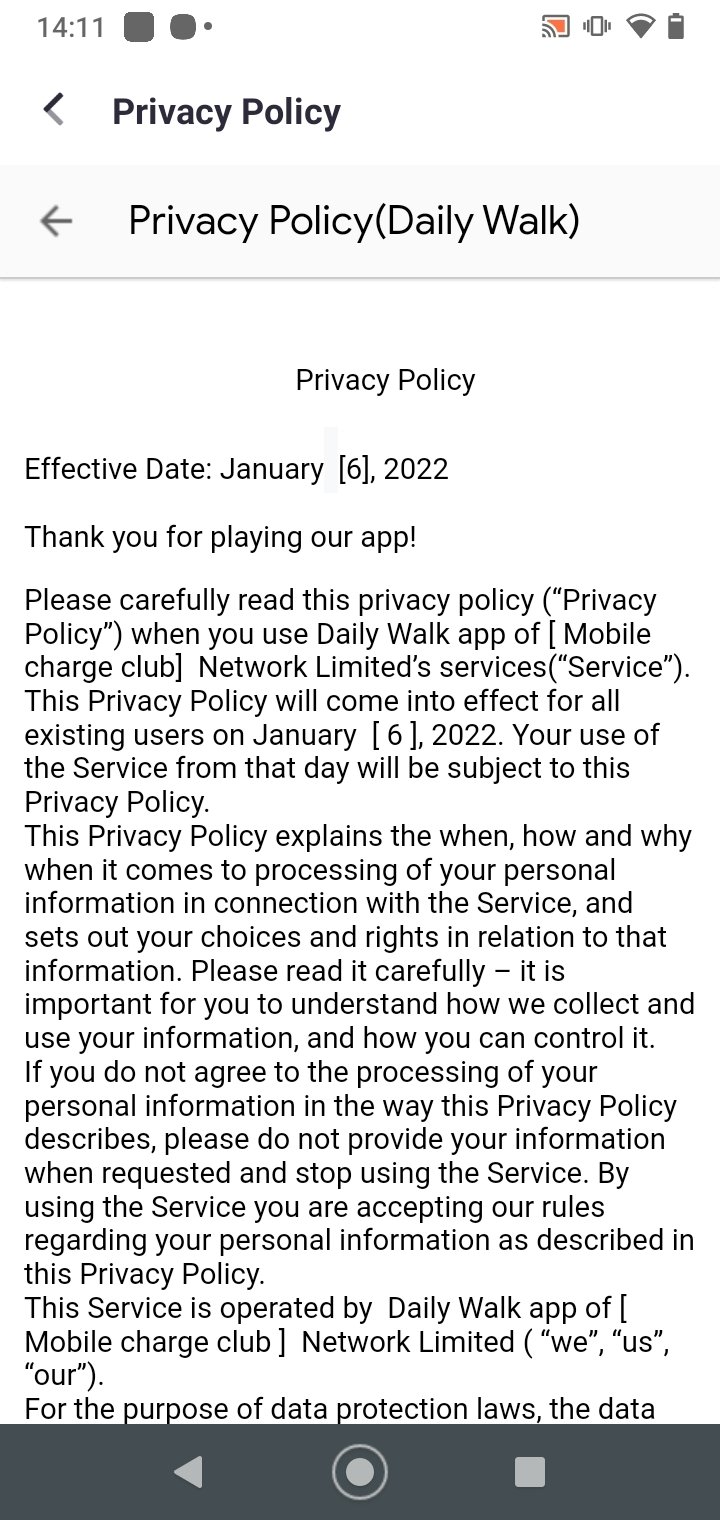A screenshot of a mobile phone displaying a privacy policy document for the app "Daily Walk" by Network Limited. The screenshot has the title "Privacy Policy" followed by the effective date: January 6th, 2022. The introductory paragraph thanks users for playing the app and urges them to carefully read the policy. It states that the privacy policy will come into effect for all existing users on January 6th, 2022, and that use of the service after this date will be governed by the terms outlined in the document.

The privacy policy explains the collection and processing of personal information, emphasizing the importance of understanding how this information is used and how users can control it. It instructs users to stop using the service and avoid providing personal information if they disagree with the policy terms. Acceptance of the privacy policy is a prerequisite for using the service.

The policy document further specifies that the service is operated by "Daily Walk App" under "Mobile Charge Club" and Network Limited, collectively referred to as "we," "us," and "our" for the purposes of data protection laws. The text ends abruptly at the bottom of the screenshot, indicating that more information is available but not visible in this particular image.